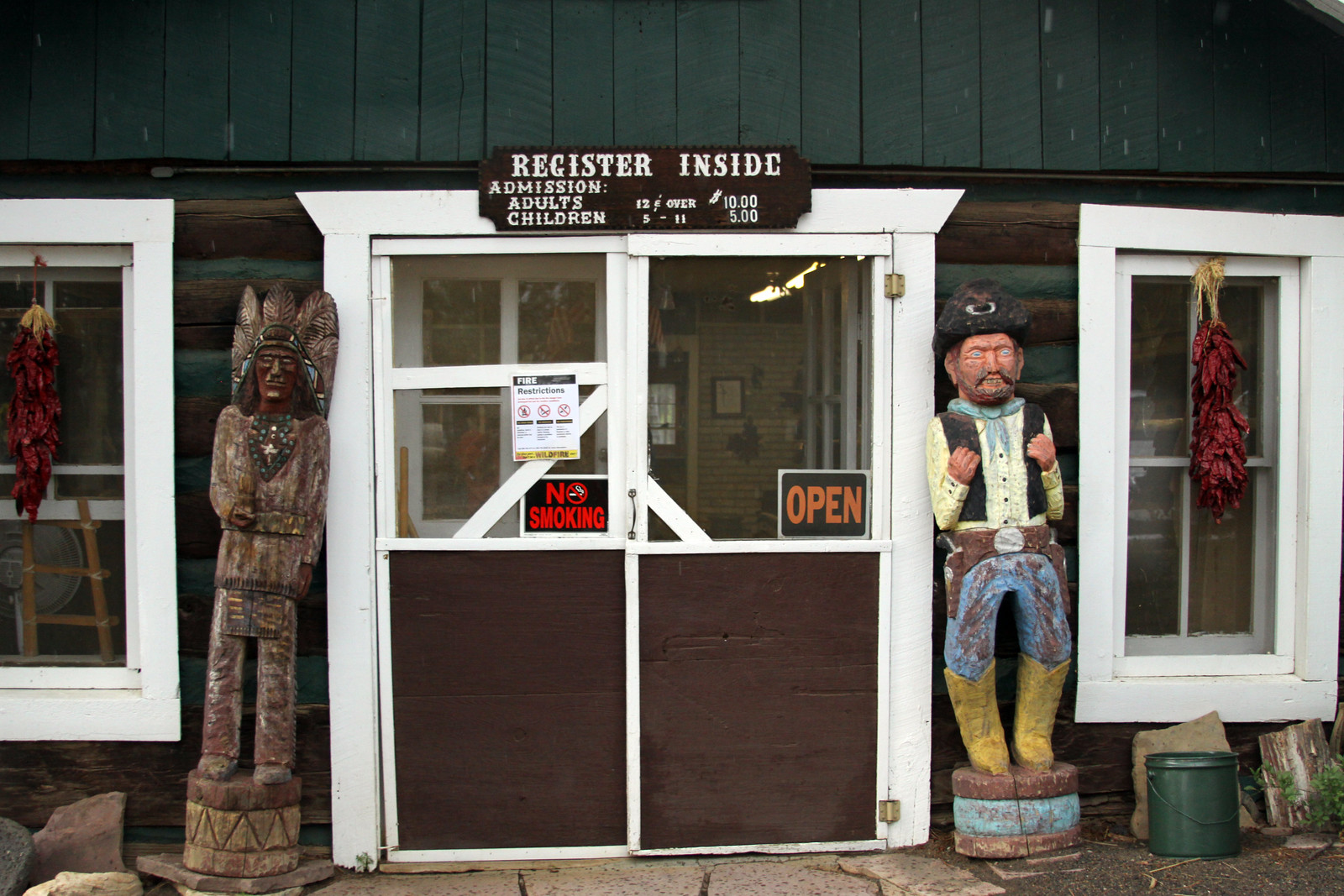The image depicts the entrance to a park or museum featuring a green wooden canopy atop a log-walled building. Central to the entrance are double doors, with the upper halves made of glass and the lower halves of brown wood, flanked by windows. Prominent on the doors are signs reading "Register Inside" and "Admission," detailing that adult entry (12 and over) costs $10, while children's entry (ages 5 to 11) is $5. There's no mention of admission fees for children aged 0 to 4, implying they might enter for free. A "No Smoking" sign and an "Open" sign are also visible on the doors.

Standing to the left of the door is a wooden Indian statue, and to the right, a wooden cowboy statue. The ground in front of the entrance is rock-strewn, and additional details include a green bucket, a piece of wood, and a tree stump near the statues. Red chili peppers hang in front of the windows, adding a splash of color to the rustic scene. Despite the open sign, there are no people visible in or around the booth.